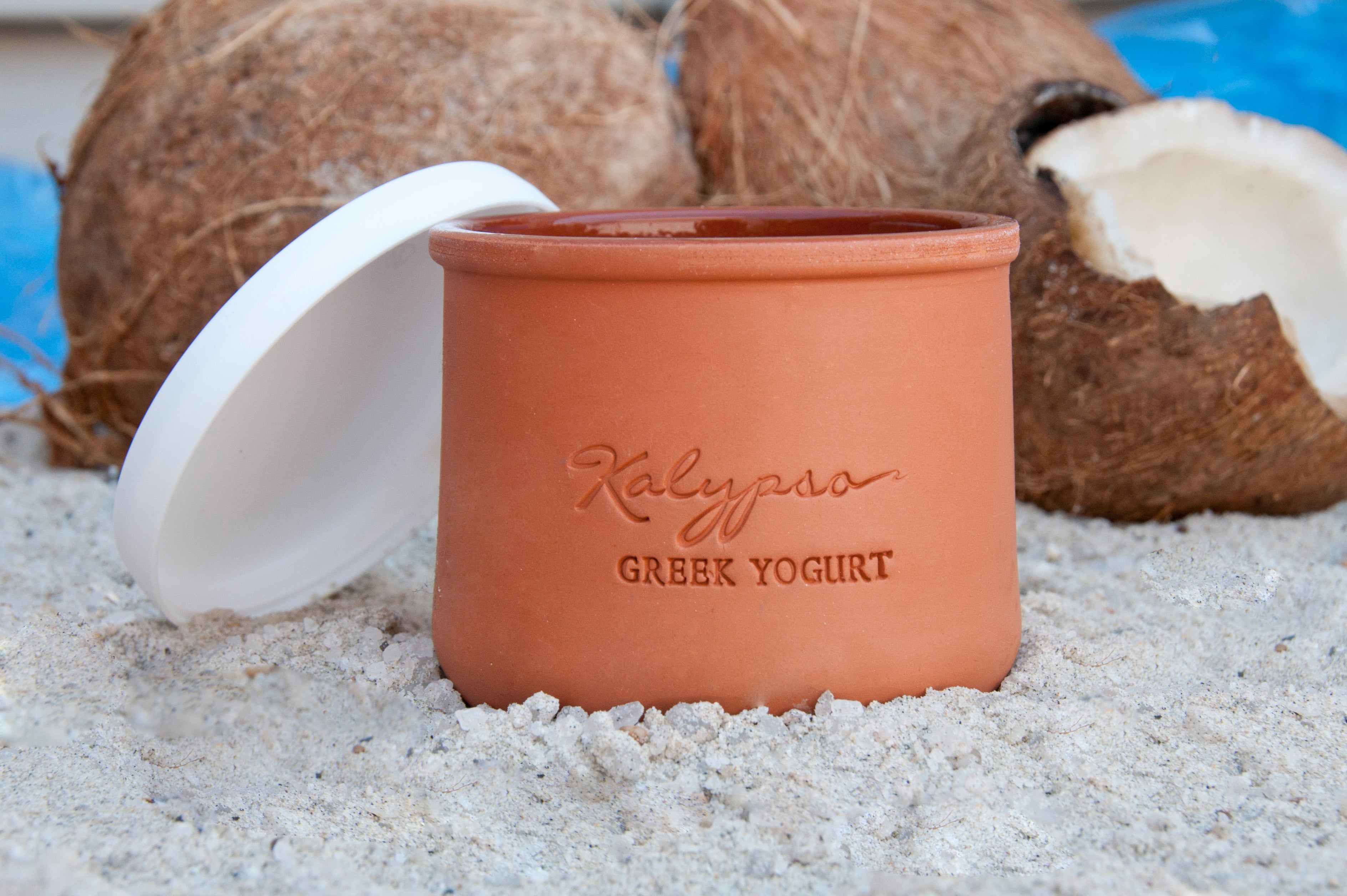The image features a small, round, terracotta-like ceramic jar with a white lid propped against its left side, resting on fine white sand scattered with small white stones. The jar itself is a light orange hue with a polished dark red interior. Enscribed in cursive on the front of the jar is the brand name "KALYPSA," with "Greek Yogurt" printed below in a more straightforward font. In the background, there are three coconuts: two whole on the left and center, and one cracked open on the right, exposing its white flesh. Behind the coconuts, a stream of vibrant blue water adds a tranquil touch to the scene, though it appears slightly blurred compared to the sharply focused ceramic jar in the foreground.